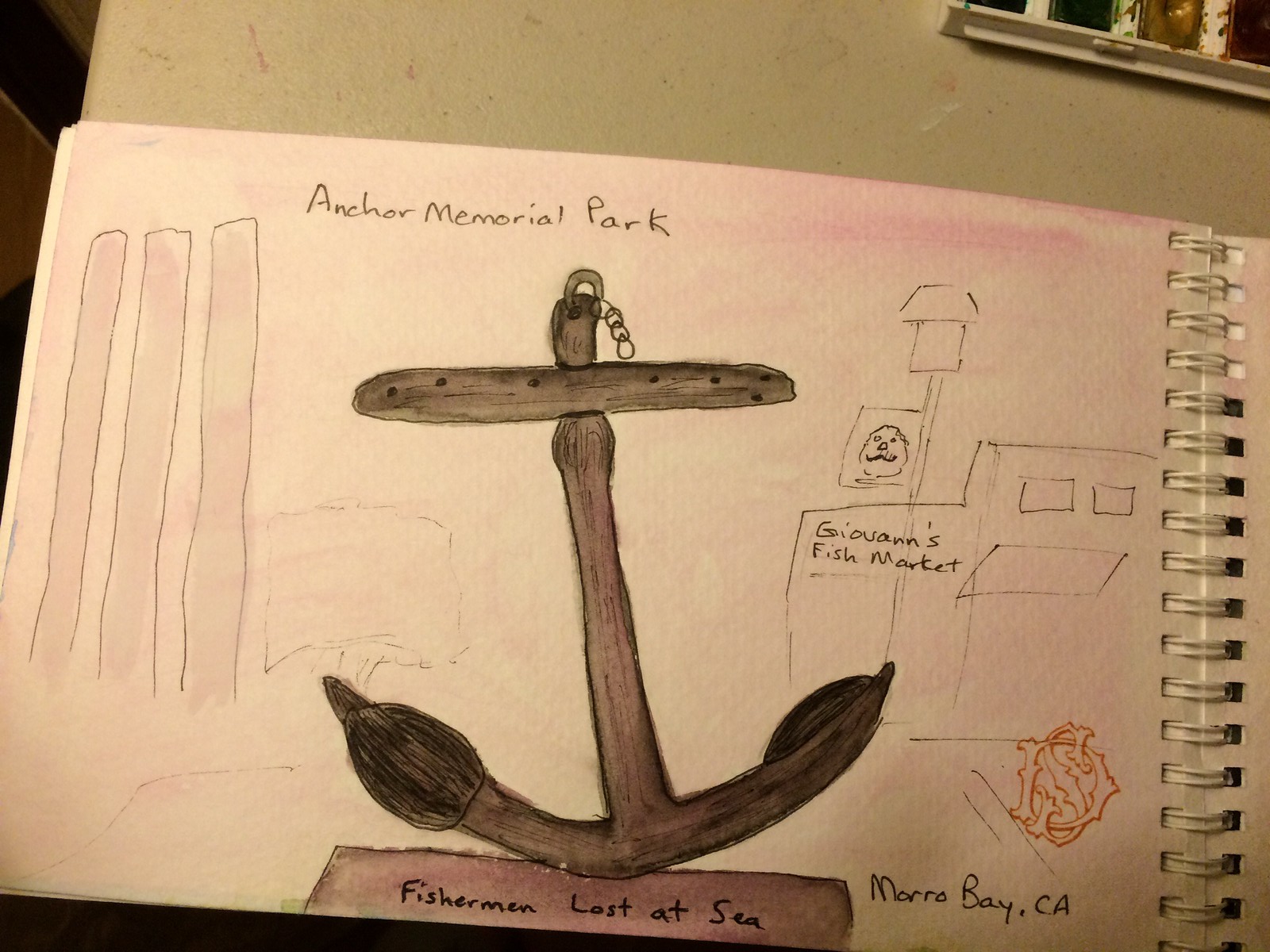This photo captures an open sketch pad laid flat on an off-white table. The sketch pad is opened to a detailed drawing. At the top of the page, the title "Anchor Memorial Park" is meticulously inscribed. Dominating the center is an intricately drawn dark gray anchor, symbolizing the memorial theme. Below the anchor, the poignant phrase "Fisherman Lost at Sea" is carefully written, adding emotional depth to the artwork. To the right side of the page, there is a depiction of a store with a sign reading "Giovanni's Fish Market" accompanied by the location "Morrow Bay, California" underneath. In the upper right-hand corner of the image, part of a paint tray is visible, giving a glimpse into the artistic process behind the sketch.